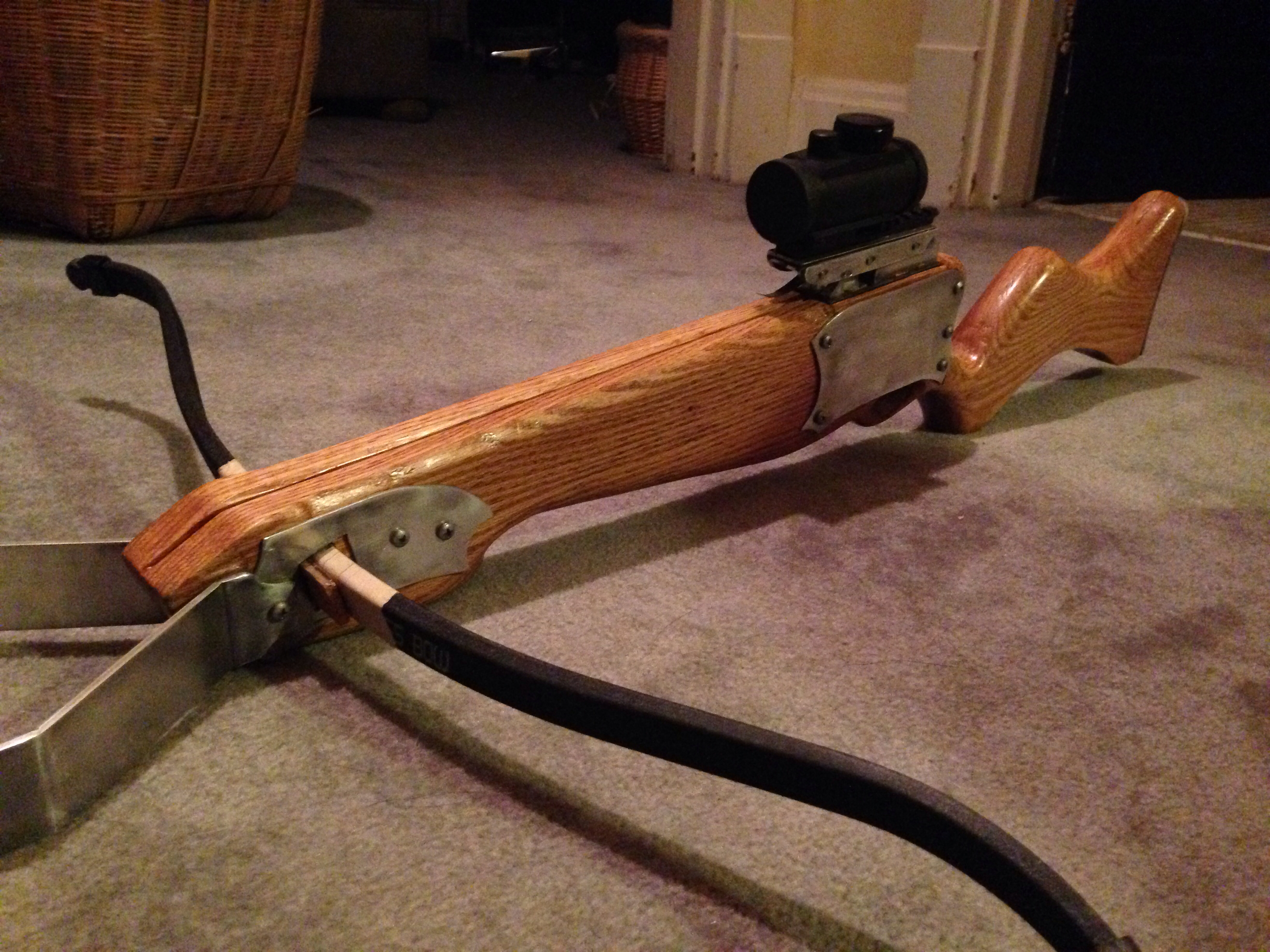In this horizontally oriented photograph, a modern wooden crossbow dominates the center, oriented diagonally toward the bottom left. The crossbow, rustic yet sophisticated, features a mix of materials: a polished wooden stock shaped like a rifle's butt, complete with intricate contours, and a sleek black scope mounted on top, reminiscent of those on sniper rifles. The front bow section is marked by two outward-extending black limbs where the string would attach, accompanied by metal prongs secured firmly into the wooden frame. The background comprises a grayish, possibly dirty carpet covering the floor, adding a rugged texture to the scene. Surrounding objects include a woven wicker basket in the top left corner and another basket closer to the center of the top edge, suggesting a cozy yet cluttered interior space. Additionally, the setting reveals part of a wall near the middle top and an open doorway to another room on the top right, hinting at a domestic backdrop to this intriguing piece of weaponry.